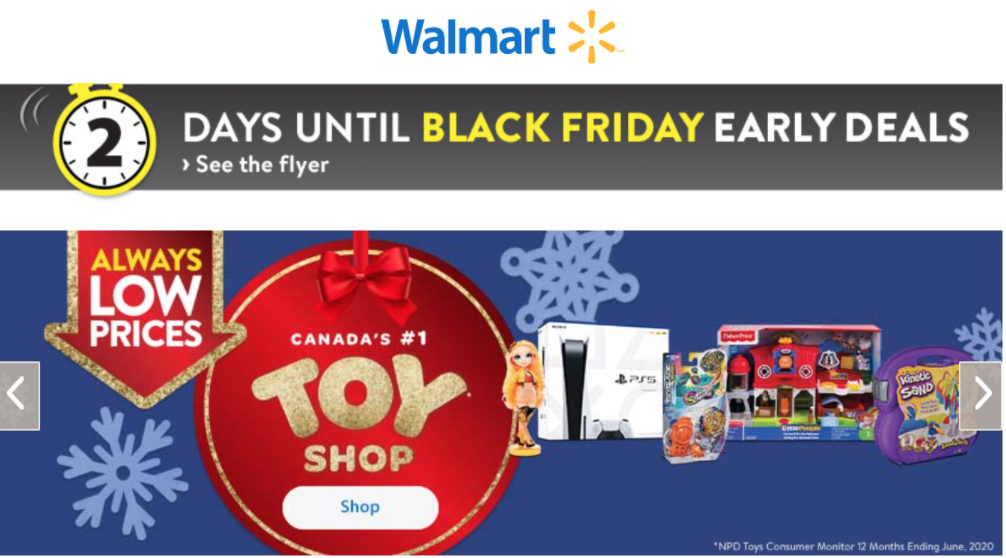A screenshot featuring a vibrant blue background prominently displays a countdown stating "Two Days Until Black Friday" alongside yellow text announcing "Early Deals". At the top of the image, the Walmart logo and its tagline, "Always Low Prices. Always." stand out in yellow. An oval-shaped white button with "Shop" written in blue is also visible. The screenshot highlights Walmart as "Canada's Number One Toy Shop" and showcases several toys, including a doll, a PlayStation 5, a toy ramp with a car, a Fisher-Price house, and a purple case labeled "Kinetic Sand". At the bottom of the image, a star icon accompanied by the text "NPD Toys Consumer Monitor" is displayed. The flyer invite to "See the Flyer" is also featured, guiding consumers to more deals.